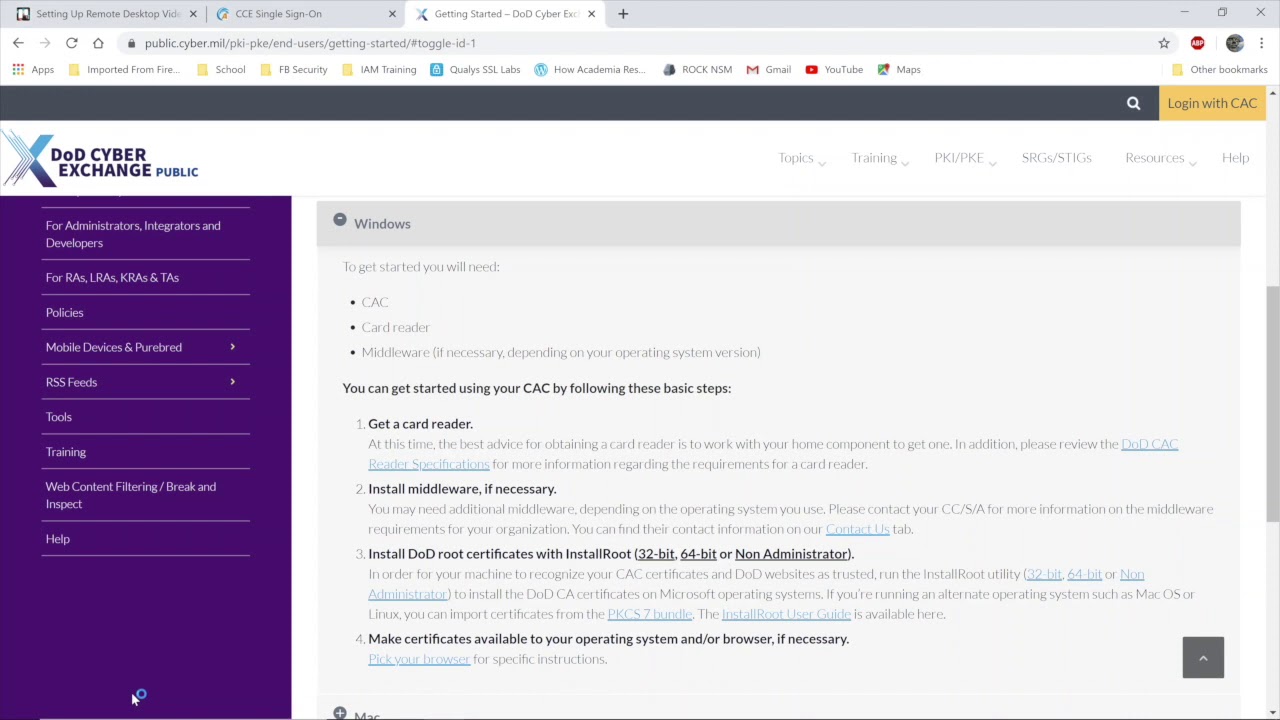**Descriptive Caption:**

The image showcases the DOD Cyber Exchange Public web page tailored for Administrators, Integrators, and Developers. On the left-hand side, there is a comprehensive menu presented in white text within a purple box, listing categories such as RAs, IRAs, KRAs, TAs, Policies, Mobile Devices, PureBread, RSS Feeds, Tools, Training, Web Content Filtering, Break and Inspect, and Help. 

At the very top right-hand side of the page, several key sections are highlighted: Topics, Training, PKE, PKI, SRG, STIGS, Resources, and Windows. 

Underneath the Windows section, guidance is provided for getting started with the site. Users will need a CAC, a Card Reader, and possibly Middleware, contingent on their operating system version. The instructions advise users to procure a card reader by coordinating with their home component and to review the DOD CAC reader specifications for detailed requirements.

The caption emphasizes the structured layout and specific guidance available on the web page, ensuring users have the necessary tools and information to access the site effectively.